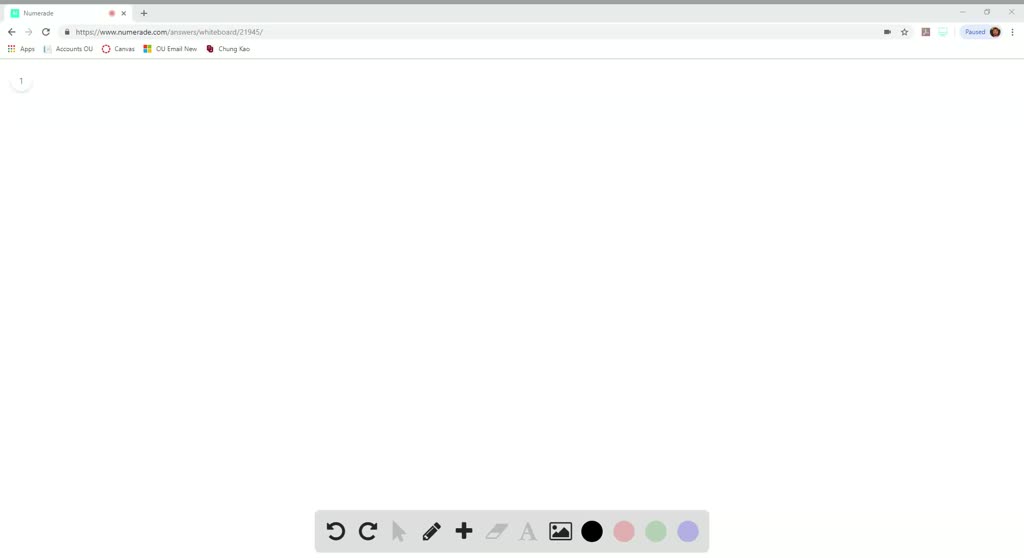The image depicts a partially loaded web page with a detailed header and footer. At the top, a dark solid gray line stretches horizontally across the page. Beneath this, there is a larger gray rectangle encompassing a smaller white rectangle positioned to the left. Inside the white rectangle, there's an aqua green square featuring indistinct black text and accompanied by a red dot and a black 'X' next to it.

Below the gray rectangle, a navigation bar showcases a dark black arrow pointing left and a gray arrow pointing right. There is also a refresh icon represented by an incomplete circle with a triangle at its end. Additional small black text is visible, including the word "apps," but most of the writing is illegible due to its size.

At the bottom of the page, a gray square contains several icons: a half-circle with a triangle tip on both the left and right sides, a pencil, a plus sign, a square with a mountain illustration inside, a solid dark black button, and three light-colored buttons (red, green, and blue).